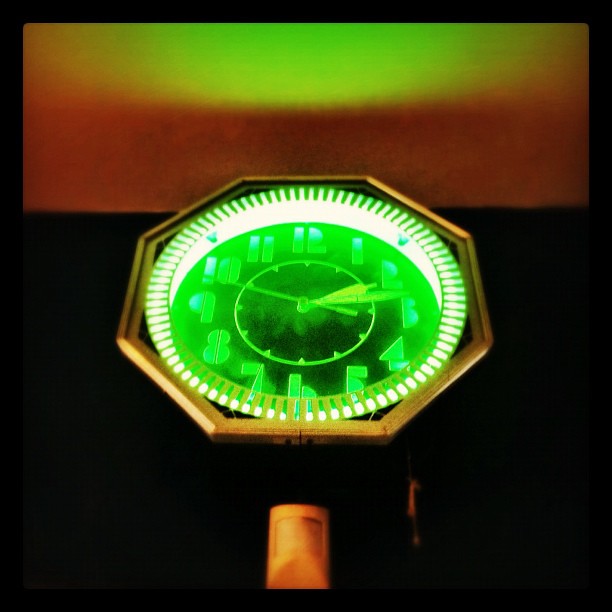The photograph is a highly detailed, colorful image featuring a luxurious timepiece. Central to the composition is an octagonal, golden watch case, which holds the focal point of the image—a luminous green watch dial. The dial is striking with its fluorescent green glow, bordered by a white section followed by alternating green and white lines. The numbers and other markings on the dial share the same greenish hue, enhancing the overall luminescence. 

Below the watch dial, the photograph shifts to a black background, punctuated by a small, orangish handle before it transitions back to black. Above the dial, there is a border in orange and fluorescent green, which may be illuminated by a light source, casting an intricate interplay of colors upon the timepiece. The vibrant hues and meticulous detailing suggest that the watch dial is the main component of the photograph, drawing the viewer's attention to its elegant design and craftsmanship.